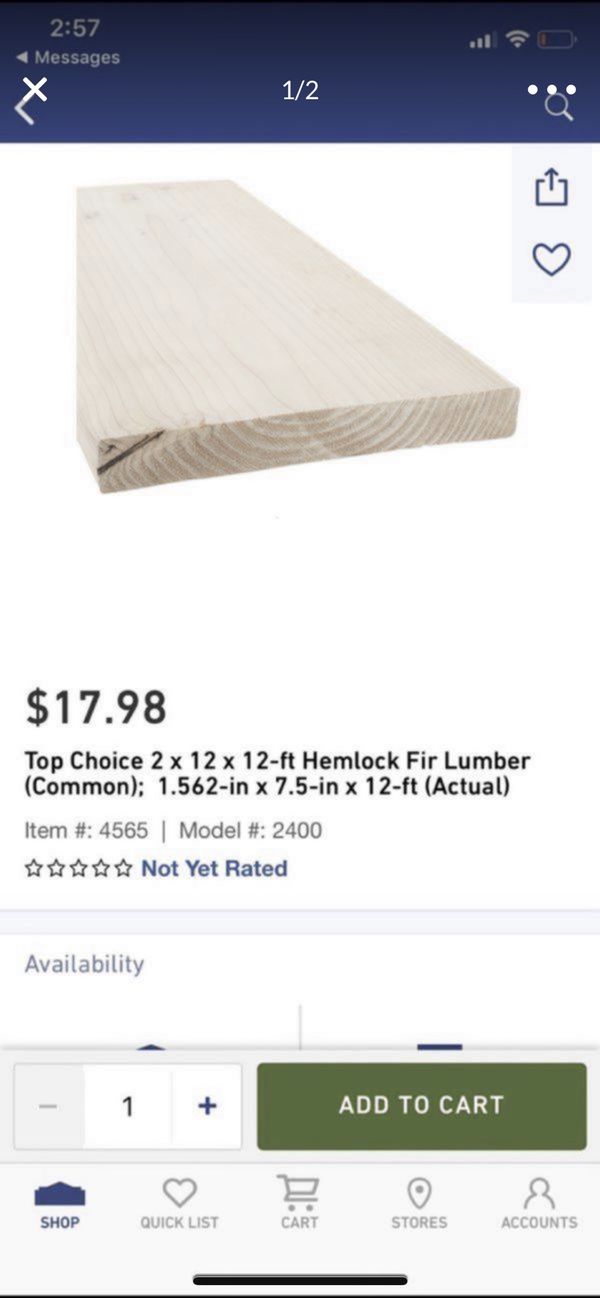The image features a detailed online product listing for a piece of lumber. At the top of the screen, the time is displayed as 2:57, with a Wi-Fi icon to its right. The background transitions from black at the top to dark blue beneath the icons. 

Below this gradient, the main section of the image is set against a white background, showcasing the piece of lumber from a front edge and top view. To the right of the lumber image, there are print and heart icons. The price, $17.98, is prominently displayed, followed by the product description "Top Choice 2x12x12 feet Hemlock FIR lumber." The item number 4565 and model number 2400 are listed below, with a note that the product is "not yet rated." 

Further down, the term "availability" is noted, followed by the quantity selector set at 1, featuring a minus sign to decrease and a plus sign to increase the quantity. To the right of this, a green rectangle with white text invites the user to "add to cart."

At the bottom of the image, a navigation bar for the application or webpage is shown on a light gray background. The options, from left to right, are: "Shop" (highlighted in dark blue), "Quick List," "Cart," "Stores," and "Account." Finally, a black bar is visible at the very bottom center of the image.